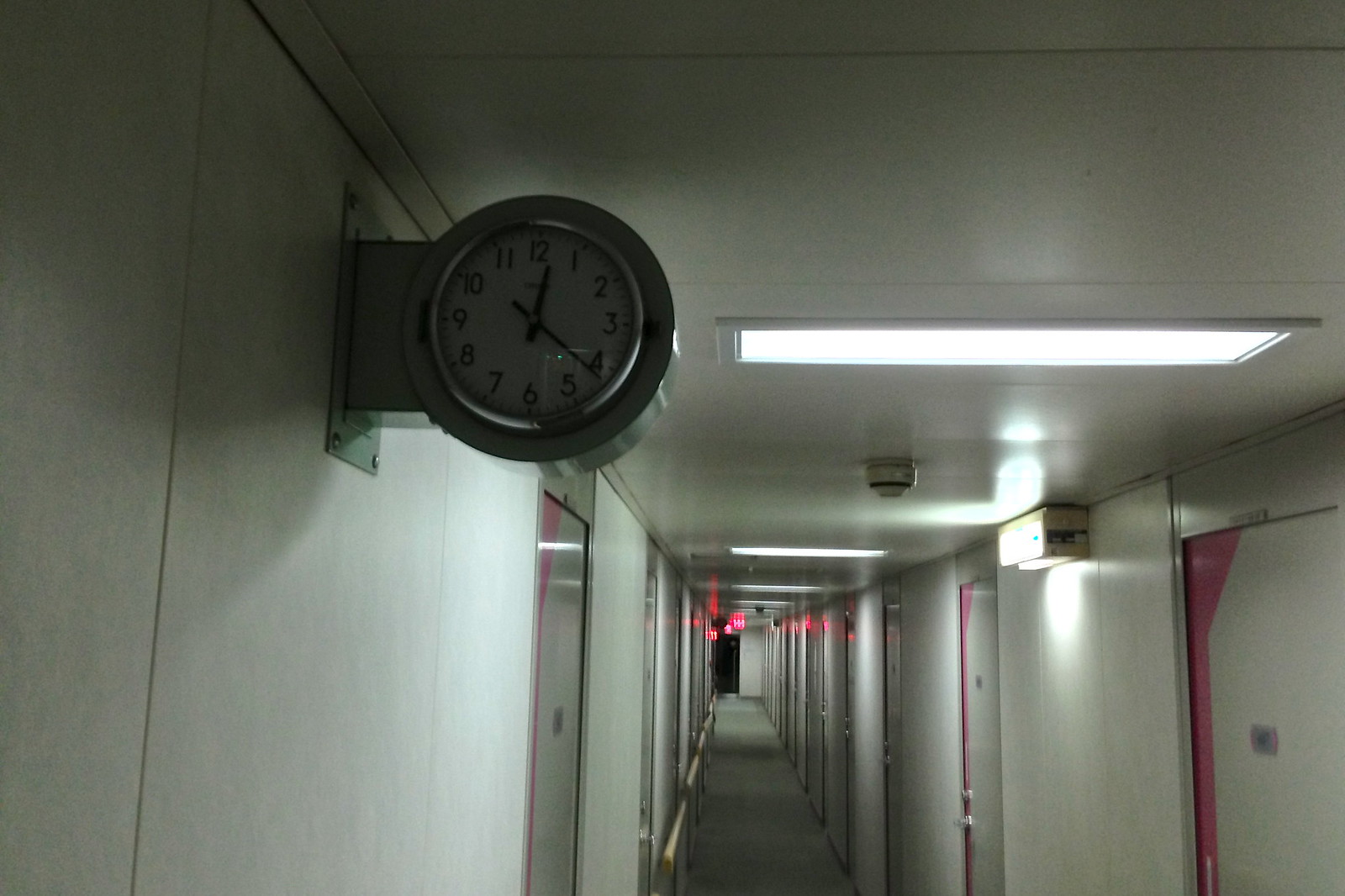The image depicts a long, vacant hallway, presumably in an office building, characterized by its narrow width and numerous doors lining both sides. The walls and doors are predominantly white, with the doors featuring a subtle pink accent. Fluorescent lights are fixed to the ceiling, providing stark illumination, while an air conditioning unit is visible on the right side. At the far end of the hallway, an illuminated exit sign emits a red glow, partially reflecting off the nearby doors.

The most prominent feature in the foreground is a round wall clock protruding from the left side, near the ceiling. The clock is mounted on a rectangular bracket bolted to the wall. Its white face displays Arabic numerals, and it has black hour and minute hands. The time indicated is between 12:20 and 12:25.